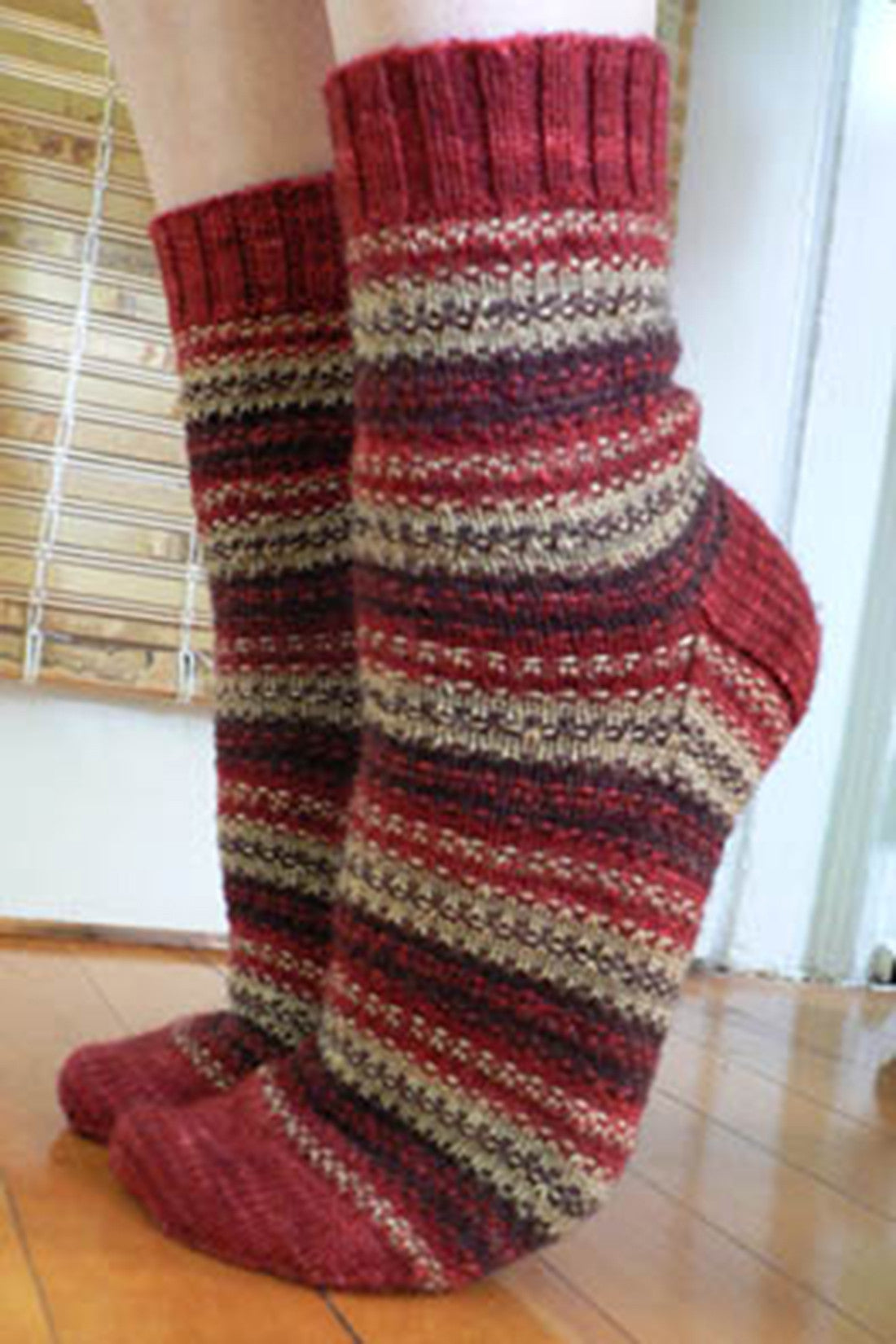The photograph captures a close-up of a pair of feet extended upward as the person stands on their tiptoes, emphasizing the cozy and snug look of their woolen socks. The socks are predominantly red with distinct black, red, and brown horizontal stripes running all the way up. The toes, heel, and ribbed cuffs are reinforced with a thicker red material, highlighting the robust construction suitable for colder weather. The skin tone of the person is light, suggesting they might be Caucasian. They are standing on a highly polished, light brown wooden floor, characterized by tiny black gaps between the panels. In the background, a white wall is visible along with a window covered by a unique wooden curtain made of panels lashed together with white string, creating an earthy, rustic ambiance.